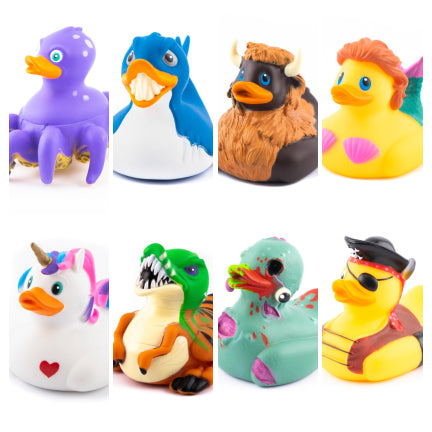This image showcases a whimsical collection of eight themed rubber ducks arranged in four rows, with two ducks per row, set against a white background. In the top row, the first duck resembles a purple octopus with distinct tentacles, while the duck beneath it is a white unicorn with a rainbow mane and a heart on its chest. The second row features a blue and white shark-like duck sporting an array of sharp teeth, followed by a dinosaur-themed duck with a green head, jagged teeth, and a brown body. In the third row, there is a brown cow-like duck with white horns, and beneath it, a light blue zombie duck with green slime on its bill and an eyeball dangling from its socket. The final row presents a yellow mermaid duck adorned with orange hair and seashells on its chest, and at the bottom, a pirate duck complete with a pirate hat, eye patch, and a brown vest.